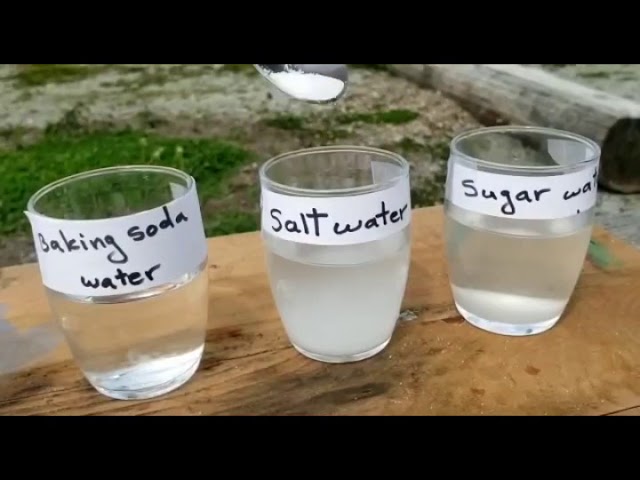In this full-color photograph taken outdoors during the daytime, likely in a park or picnic area, three transparent glasses are placed on a brown wooden table. Each glass contains a mostly clear liquid and has a white label with black handwritten text. From left to right, the labels read "Baking Soda Water," "Salt Water," and "Sugar Water." Positioned above the middle glass, there is a spoon containing a white powder, although the spoon is partially out of frame. The background features grass and soil, and there's a log visible on the upper right side. The image has black horizontal strips at the top and bottom, providing a square border to the photo.